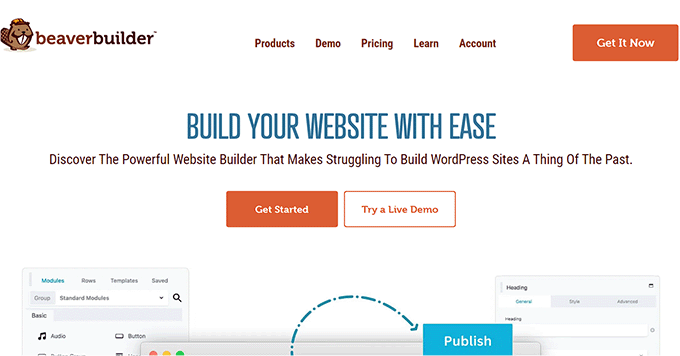The image is split into two sections. On the left side, there is an illustration of a beaver next to the text "Beaver Builder." The word "Beaver" is colored brown, while "Builder" is in black. Below this, the navigation menu displays the options "Products," "Demo," "Pricing," "Learn," and "Account," all in a cohesive brown color.

Towards the right side, an orange rectangle prominently features the call-to-action "Get It Now." Beneath it, in bold blue all-caps, is the phrase "Build Your Website with EASE." Following that, there is a descriptive tagline in black that reads, "Discover the Powerful Website Builder that Makes Struggling to Build WordPress Sites a Thing of the Past."

Further down, another orange rectangle with the label "Get Started" is positioned next to an orange-outlined rectangle that invites users to "Try a Live Demo." 

On the lower left, a gray rectangle contains some indiscernible text; the first word is blue, with the subsequent words in black text, and additional smaller, unreadable text below. To the right of this gray rectangle, there are icons of a magnifying glass, a music note, and other unclear symbols.

On the bottom right, there is an additional small gray rectangle with text; the first word on the second line is blue, with the remaining text in black. Adjacent to this is a dashed and dotted line that forms a circle and ends in an arrow pointing downwards to the right. At the bottom, there is a blue rectangle with white text that says "Publish."